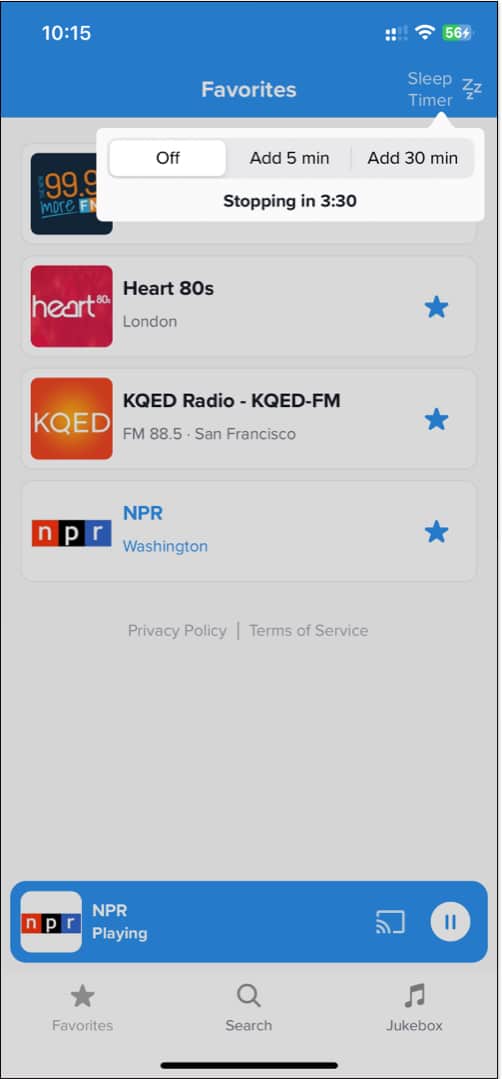This screenshot from a cell phone depicts a vertically oriented, rectangular screen. The screen features a predominantly gray background with royal blue sections at the top and bottom. 

In the top blue section, the time is displayed as "10:15" alongside battery and Wi-Fi symbols. Below this section, in the center of the screen, the word "Favorites" is prominent with "Sleep Timer" and a ZZZ icon to its right. Directly beneath the "Sleep Timer," a small white bubble is pointing upward with options like "Off," "Add 5 minutes," "Add 30 minutes," and a status indicating "Stopping in 3:30."

Further down are listings that resemble radio stations. The first listing includes a red square with the label "Heart 80s London" and a blue star icon. The next listing features an orange square labeled "KQED," followed by "KQED Radio, KQED FM, FM 88.5 San Francisco," and another blue star. The final listing at the bottom displays "NPR Washington" accompanied by a blue star.

At the very bottom of the screen, there is a large blue rectangle spanning the width of the phone with the NPR logo on the left. It reads "NPR Playing," followed by a rectangular icon, possibly representing a radio, and a white stop button with two vertical lines inside a circle to the right.